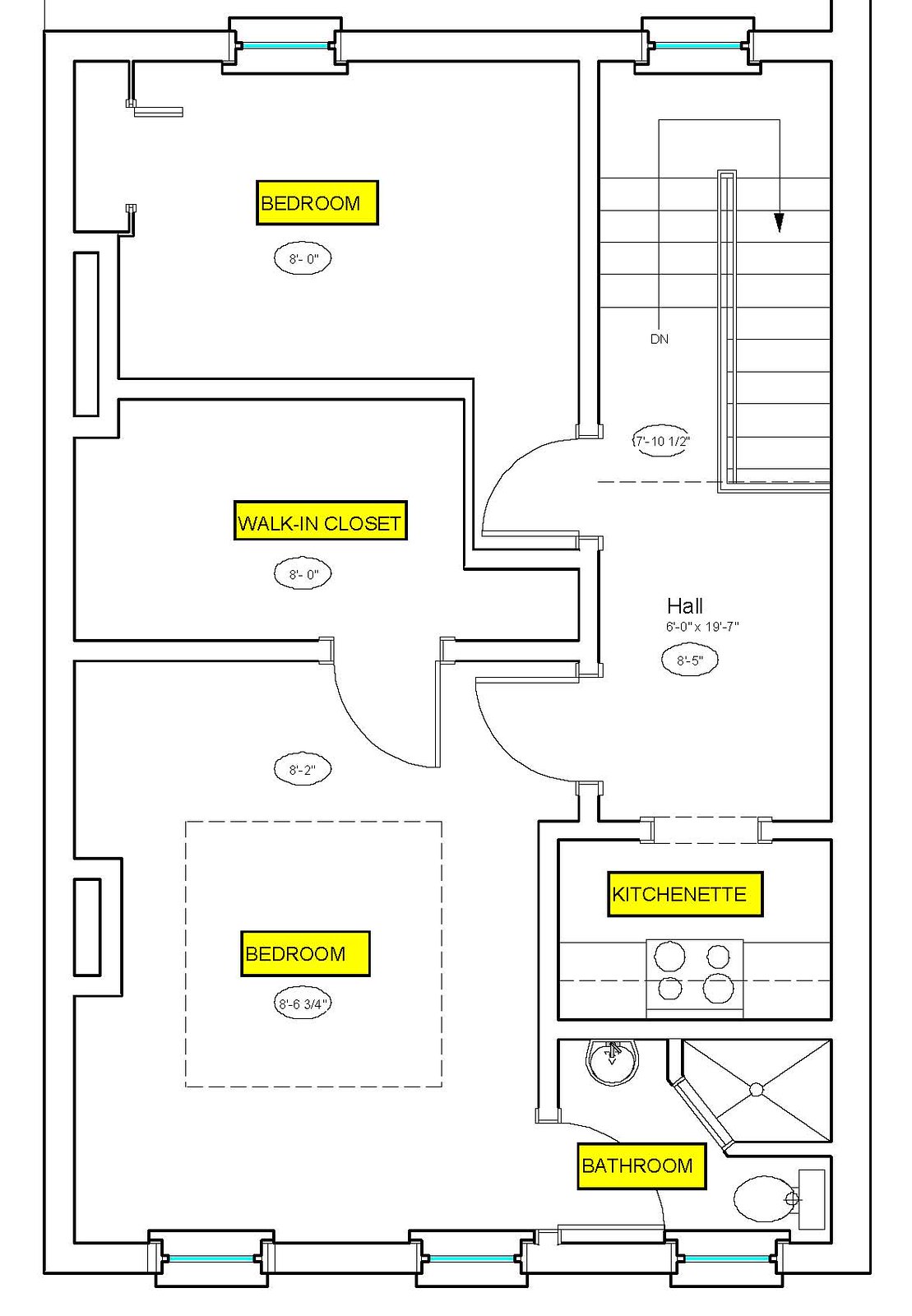The image is a detailed blueprint diagram of a home's interior layout. At the bottom of the diagram, three horizontal rectangular shapes are depicted, each intersected by a blue line at the center. Among these shapes, one yellow rectangle is labeled "Bathroom," featuring a detailed sketch of the space. Above the bathroom, another yellow rectangular section is labeled "Kitchenette" in black text with a black outline. Adjacent to these areas, to the left, is the "Bedroom," represented by a gray dotted line forming a square. Above the bedroom is the "Walk-in Closet."

To the right of the closet, the diagram notes "HAL" along with specific measurements. In the top left corner of the blueprint, another "Bedroom" is shown with its layout and spatial structure indicated. To the right of this bedroom, a series of gray lines appear; some run horizontally while others go vertically in the center. One distinctive gray line, marked "DN," traverses vertically and horizontally before dropping downwards, ending with a black arrow.

At the top of the diagram, two additional rectangular shapes are enclosed within the outer boundary, each featuring horizontal blue lines. This comprehensive layout completes the illustrated blueprint of the home's interior spaces.